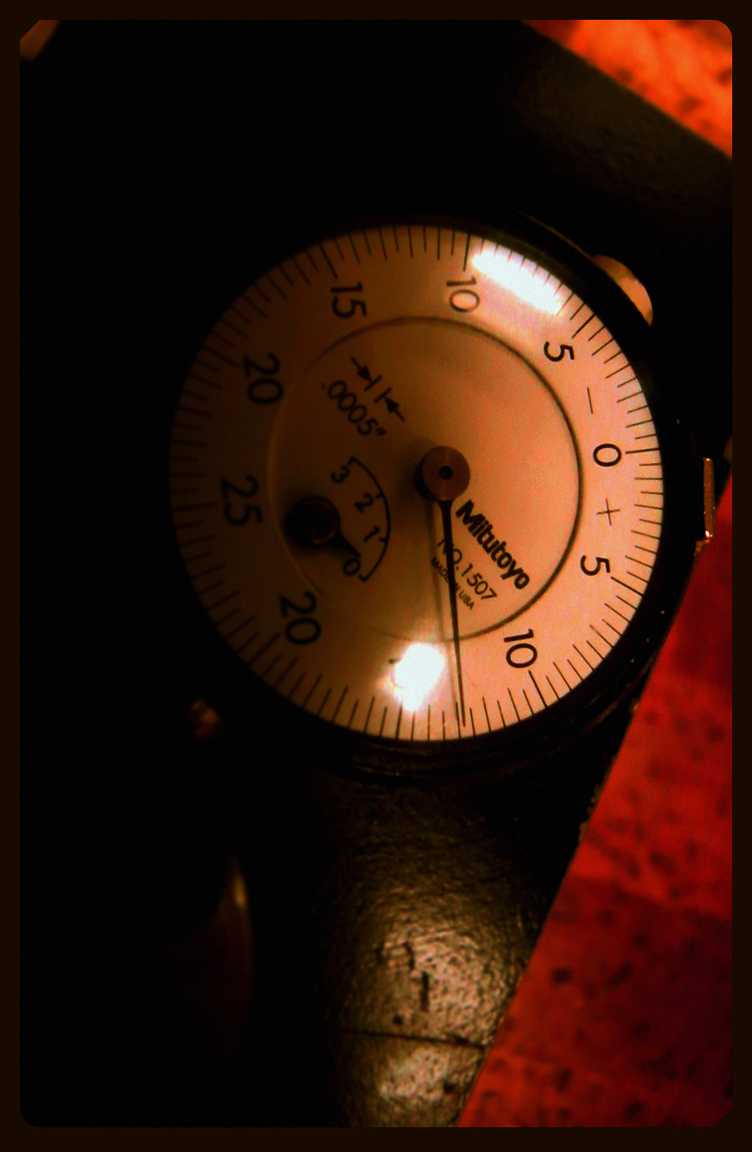The image is a close-up view of a pressure gauge, featuring a white dial with a black rim and notches encircling its perimeter. The gauge displays both positive and negative pressure values, with numbers clearly marked around the dial. The zero point on the dial is situated towards the right corner, with a 25 on the far left side. To the right of the zero, the dial shows a +5 at a long notch, followed by smaller notches leading up to a +10, +15, +20, and +25 in a sequential manner. Continuing in a counterclockwise direction from the +25, the numbers decrease symmetrically through +20, +15, +10, and +5, until reaching the left-side zero point and then transitioning to negative values. The precise arrangement of notches and numbers allows for detailed monitoring of the pressurized system. The orientation and meticulous markings suggest that it might be used in a technical or industrial setting, though it does not appear to be an oxygen-specific gauge.